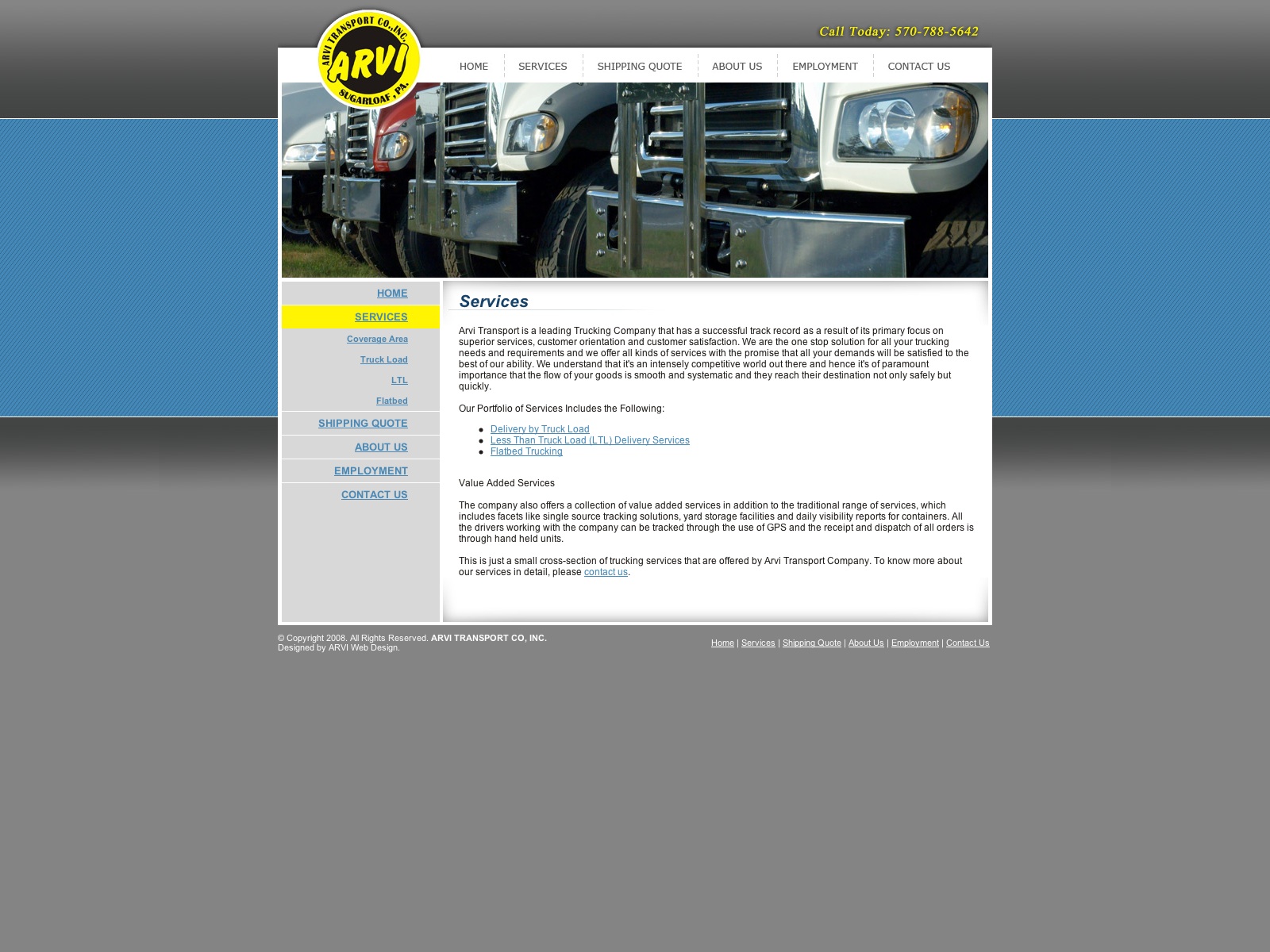This image features a professional and cleanly designed website for a car and truck repair company. The website is set against a meticulously structured background composed of horizontal borders. At the top, a thin gray border is followed by a larger blue border approximately two and a half to three times its size. This is succeeded by an even larger gray border. These borders collectively form an elegant frame for the content within.

The primary content area is a square section characterized by a pristine white background. Dominating the top is the company's logo: a distinct yellow circle encasing a black circle with the letters "ARVI" prominently displayed in yellow across the black center, offering a stark contrast and brand recognition.

A horizontal white navigation bar is situated below the logo, featuring clickable sections such as "Home," "Services," "Shipping Quote," "About Us," "Environment," and "Contact Us." Directly beneath this, a vibrant image of multiple trucks lined up side-by-side stretches horizontally, visually connecting to the company's industry focus.

On the left side of the content area is a vertical gray column with white text links, providing additional navigation options. These include "Home," "Services," a small unreadable item, "Truck Load," "LTL," "Flatbed," "Shipping Quote," "About Us," "Employment," and "Contact Us."

To the right of this column is an elongated rectangular white box labeled "Services." Below this heading is a paragraph detailing the services offered, followed by a subsection on the company’s portfolio with three clickable links for more information. The section concludes with another value-added paragraph, emphasizing the range or quality of services provided.

Overall, the structured layout and careful attention to design elements make this website not only visually appealing but also functional, reflecting the professionalism and comprehensive service offering of the car and truck repair company.